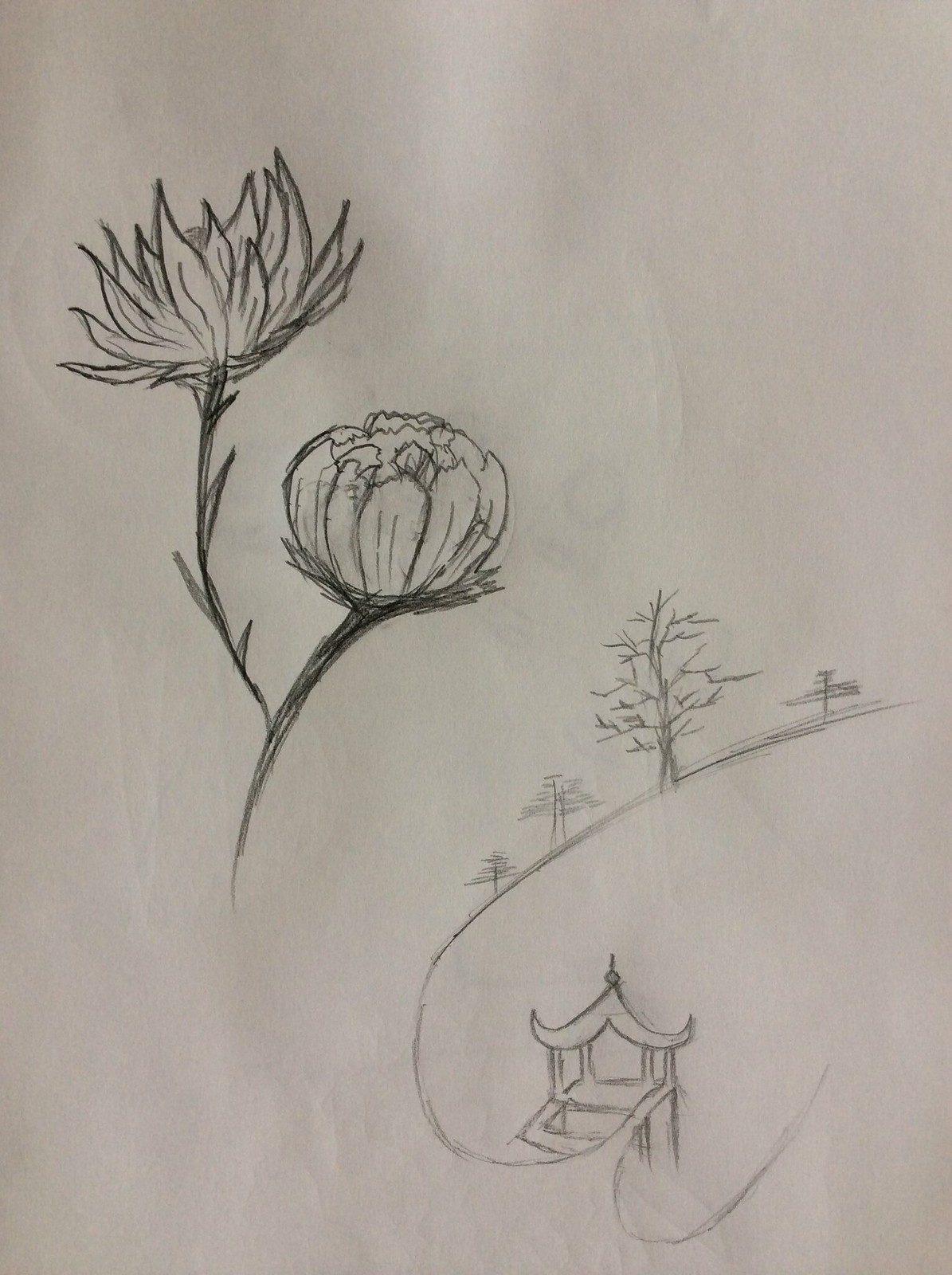On a piece of white paper, there is a detailed pencil drawing. On the left side, two different types of flowers are etched. The one furthest to the left features thorns protruding from its sides, with petals that taper to a tip before widening toward the stem. The other flower on this side has tightly closed petals, resembling a small ball. On the right side of the paper, there is an intricate etching of a gazebo, which extends into a narrow path flanked by three trees. Additionally, a direction sign is etched, guiding the viewer's eye through the scenic pathway opposite the gazebo.